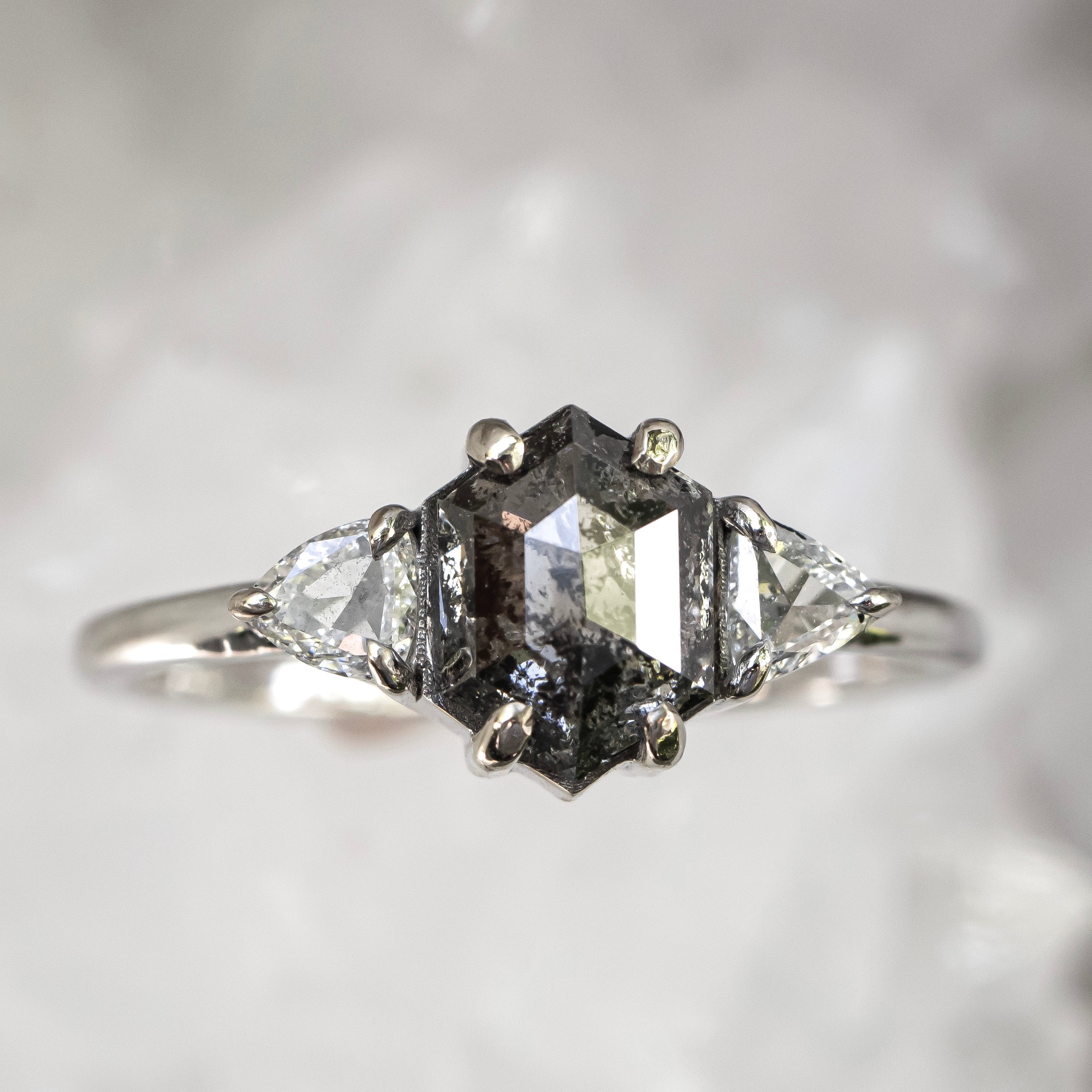This is a close-up photograph of a silver ring placed against an abstract background comprising various shades of gray. The vertical rectangular image centers on the intricate details of the ring's design. The ring features a central gemstone that is octagonal in shape, secured by four steel prongs. This central gem, possibly silverish in appearance, is flanked by two smaller, triangular-shaped diamonds, each held by three prongs. The entire band, also silver, showcases a reflective surface, which captures hints of the surrounding room and possibly the photographer. The ring is set upright using a discreet piece of blackish-brown tack against a white surface, emphasizing the sparkling, new quality of both the metal and the gems.